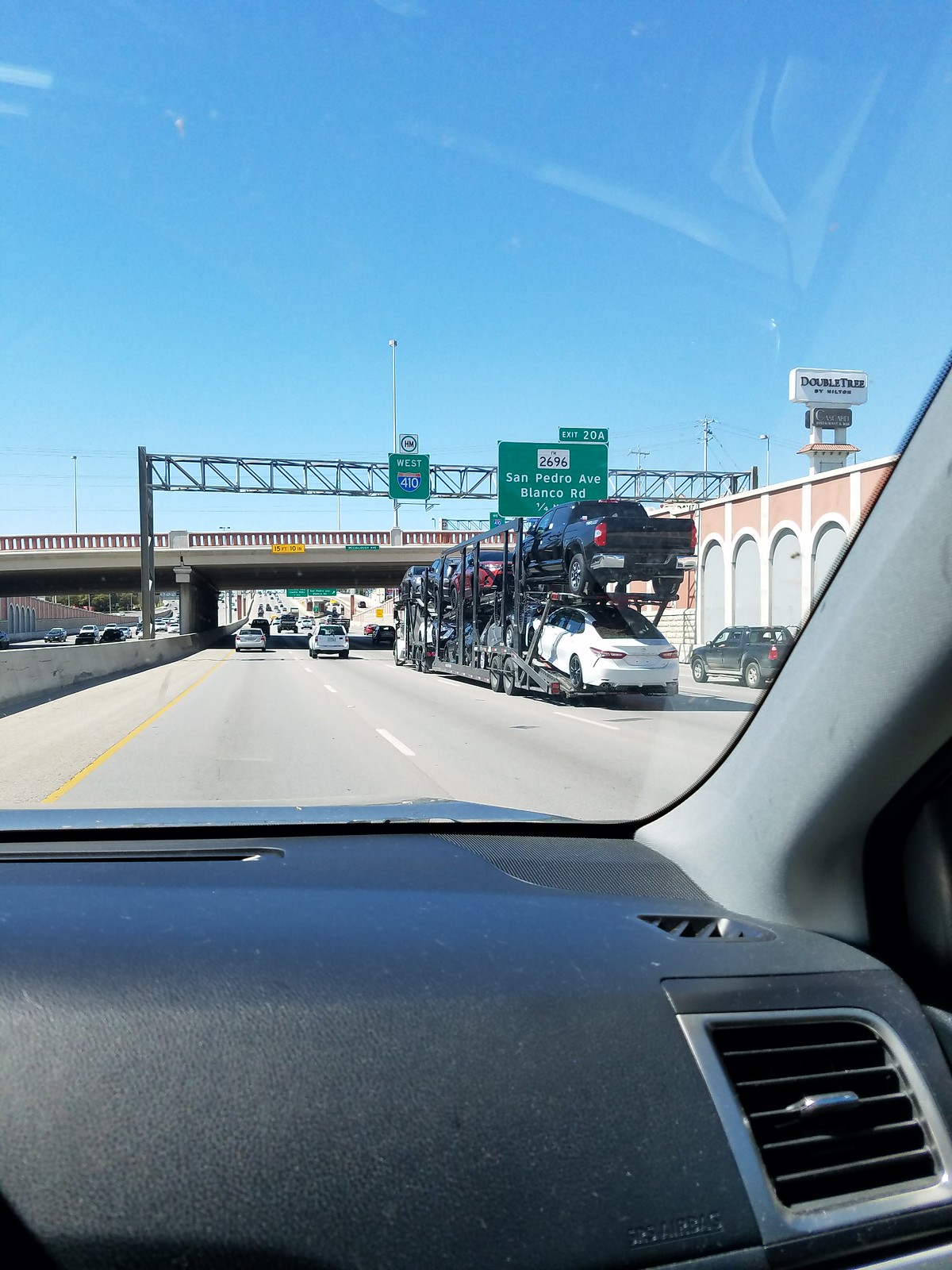This photo, taken from the passenger seat inside a black-interior car, captures the scene of an American interstate. The dashboard, air conditioning vent, and windshield are visible in the foreground. Ahead on the freeway, there is a large 18-wheeler car carrier transporting multiple vehicles on two levels. Surrounding this truck are various other vehicles, including two white cars and a black SUV to its right, while a median barricade separates the two directions of traffic. A prominent green interstate sign above the road reads "West 410," with an exit sign announcing "Exit 20A, 2696 San Pedro Avenue, Blanco Boulevard, one-fourth of a mile." Just before disappearing under an overpass, a distance sign in the upper right corner hints at a DoubleTree hotel.